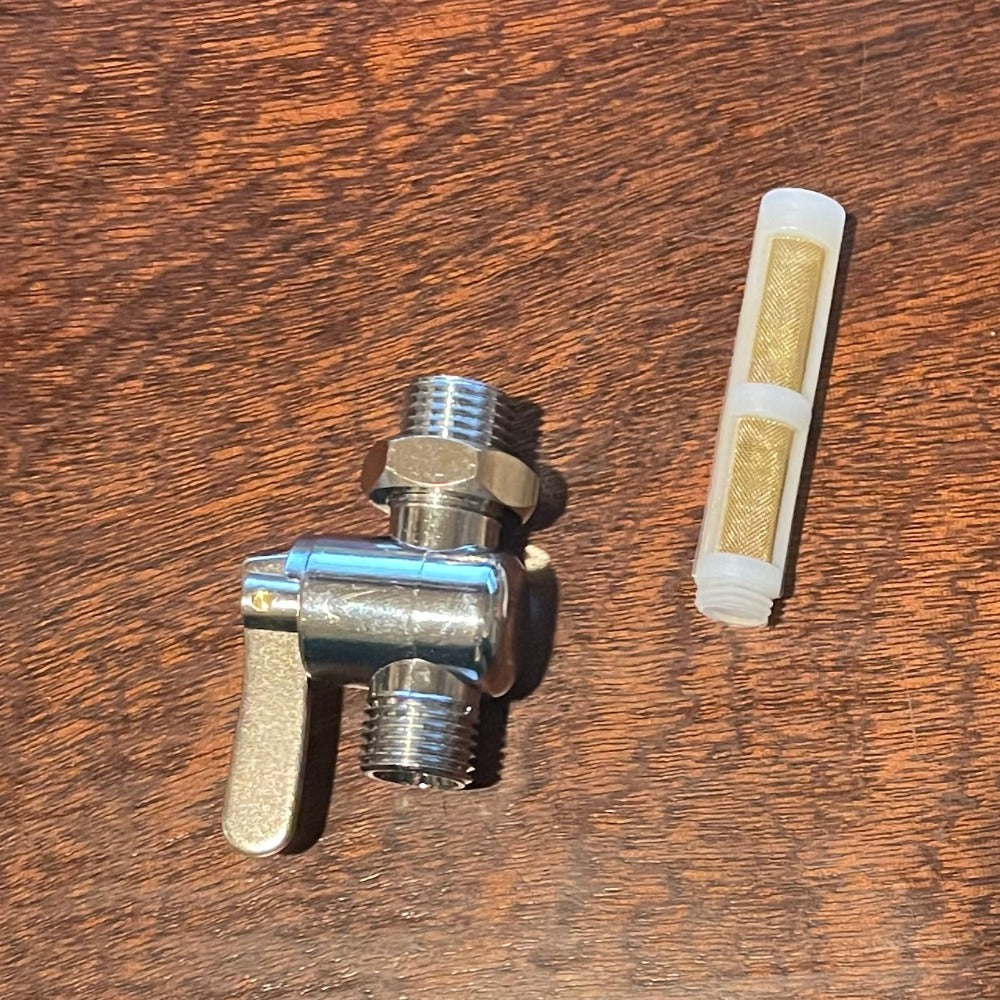This image features a shiny chrome water valve, prominently displayed on a wooden surface with a fine grain, illuminated by overhead light. The valve itself is approximately three to four inches long and has multiple threaded areas for connections: one nut around the top threaded part, another screw-on section at the bottom, and a broader central barrel. A metal handle with a gold hue is positioned on the left side, designed to rotate counterclockwise and clockwise for control. On the right side, there is a white, cylindrical plastic filter equipped with brass screening, suggesting its purpose is to be connected to the valve for water filtration or flow regulation.